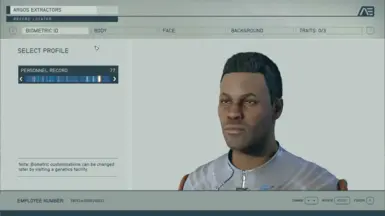This image appears to be a screenshot from a video game, possibly from a character selection or customization screen. 

In the center of the interface is a detailed profile selection menu. The left section contains several menu options, including "Profile," "Personal Record," and various colored lines, possibly representing different selection states or categories. The top gray header displays an "AE" logo on the upper right, with options labeled "Biometric ID," "Body," "Face," "Background," and "Traits." The "Biometric ID" option is currently selected, highlighted in a lighter shade.

The bottom part of the interface has a similar gray color, featuring an "Employee Number" label and several other options that are not fully legible. A solid blue line runs along the very bottom of the screen.

In the main area of the interface, a photograph of an African-American man is prominently featured on the right. He is slightly facing left and has short hair with a bit of stubble on his face. He is dressed in a futuristic gray outfit with a high collar that reaches near his neck. The outfit includes orange, futuristic-looking pads along his arms, which add a sci-fi element to his appearance. A visible zipper runs down the front of the outfit.

The overall design and futuristic elements, including the detailed character and UI components, suggest that this screen is indeed part of a complex character selection or customization process within a video game.